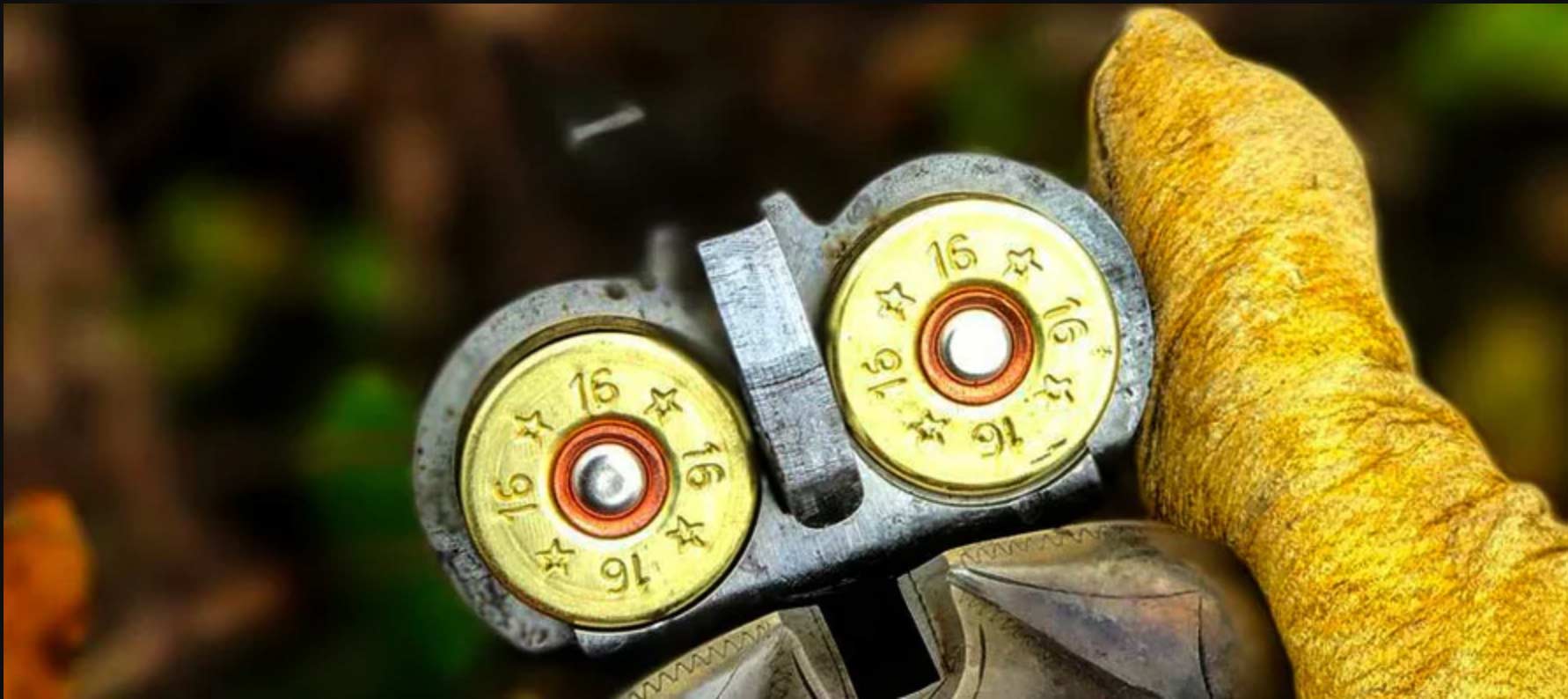This close-up photograph captures the breech of a broken-open double-barreled shotgun, specifically designed for loading. The firearm features two 16-gauge shotgun shells, identifiable by the number "16" and star engravings on their bases. The shells display a mix of colors: gold on the exterior, a silver interior encasing, and a copper-colored ring around the firing pin at their center. The metal parts of the gun exhibit a rich, blue gunmetal hue. The background is blurry, with indistinct shades of green, orange, and yellow. A gloved hand, covered in a dark mustard yellow leather glove, is seen on the right side of the image, holding the shotgun steady. The shotgun's stock, extending into the background, is made of wood.